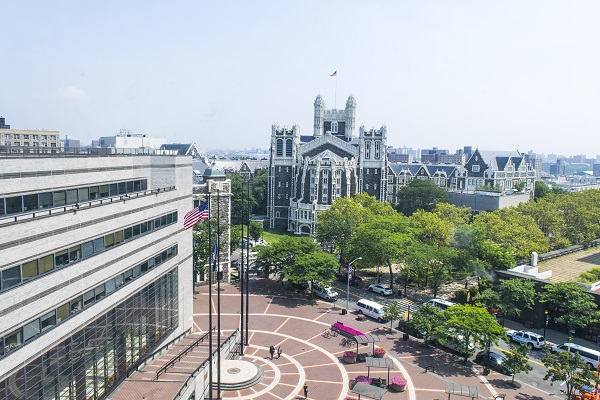The photo, taken from a perspective several stories up, showcases a sprawling city landscape dominated by a variety of architectural styles. In the background, under a hazy blue sky, stands a grand, old-style building with intricate design elements, including two prominent columns at the top, and a tall flag—possibly American—fluttering above. Surrounding this central building are clusters of green trees adding to the city's verdancy.

In the foreground, a modern multi-story building is prominent, marked by an American flag on a flagpole out front. The area below includes a brick layout with thin white lines forming concentric circles, surrounded by more buildings and a parking lot filled with parked cars. The busy streets below feature buses and cars navigating through, contributing to the vibrant urban scene.